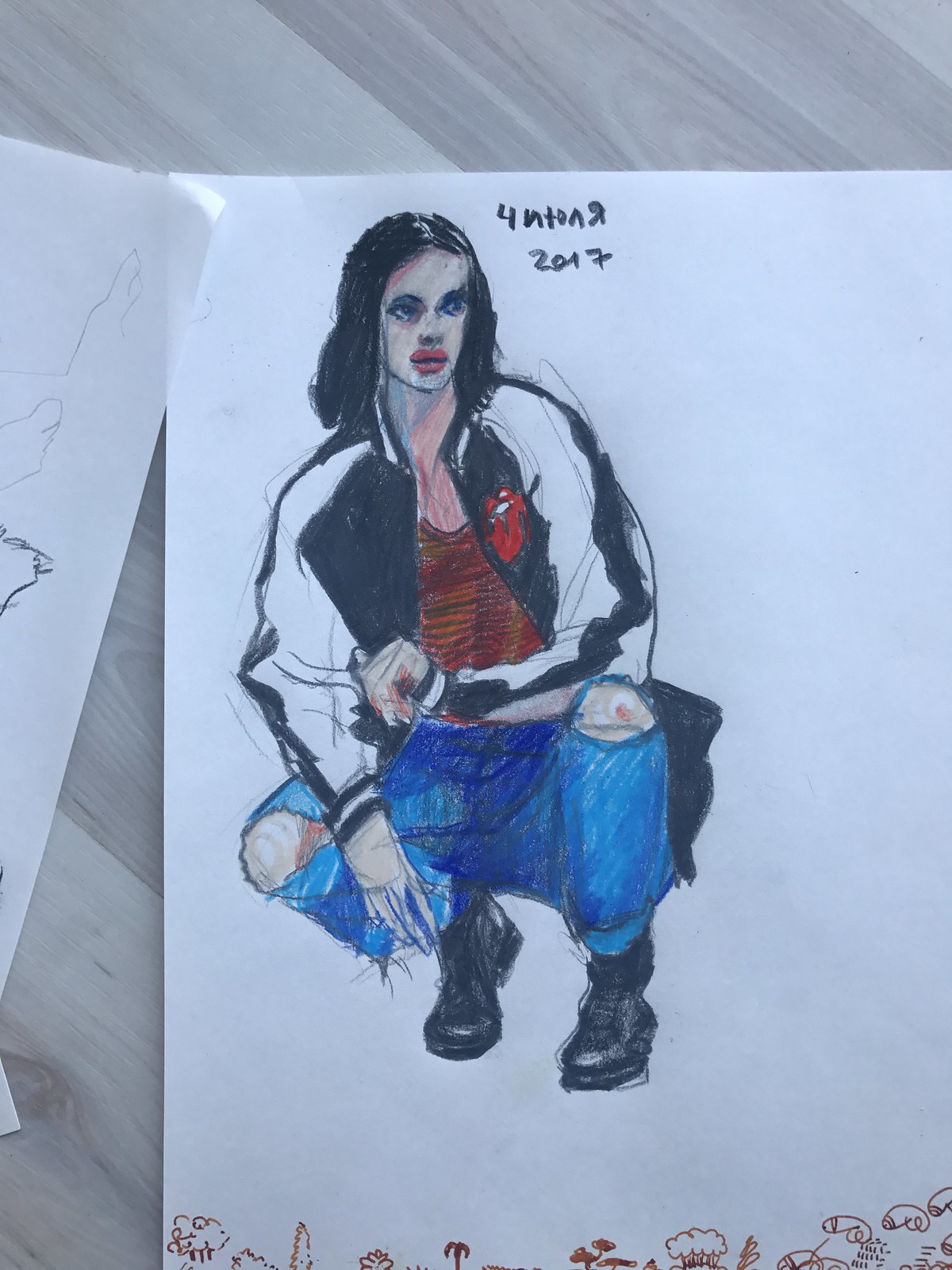The photo showcases an illustration on a piece of paper, occupying the majority of the frame. The paper rests on a white and gray wooden surface, with distinctive dark gray grain patterns visible along the left and top edges of the photo. The illustration features a white female character with shoulder-length black hair and bold red lips, her eyes accentuated with heavy makeup. Her mouth is slightly open. She is depicted wearing a black and white varsity jacket adorned with the iconic Rolling Stones logo and a low-cut, brownish-red blouse, revealing part of her neckline and chest. The girl is squatting, dressed in ripped jeans at the knees, with her hands resting on one leg, while the other hand dangles. She completes her look with black boots.

The paper also contains handwritten text reading "4NTONR2017." Below the drawing of the squatting girl, there are various small doodles, including crude sketches of penises with testicles and small tree-like figures, all done in red pen. Partially covering the top left corner of this illustration is another sheet of paper, showing some indistinct line sketches.